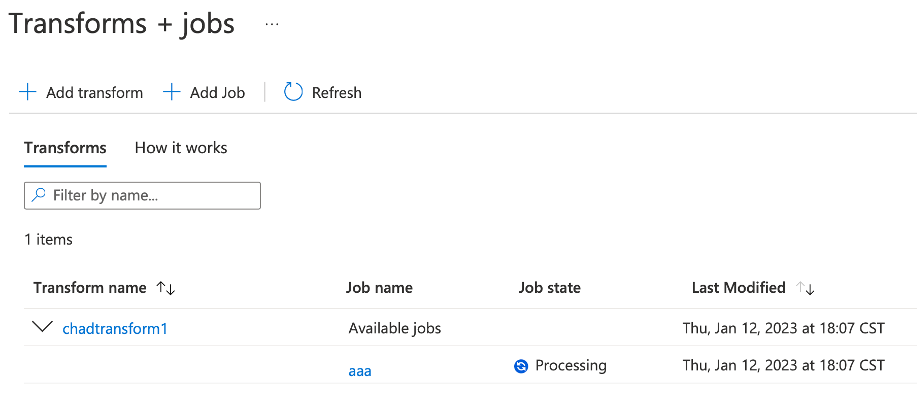Detailed Caption:

This image depicts a webpage interface primarily focused on managing transforms and jobs. At the top, there are three prominent buttons labeled "Add Transforms," "Add Jobs," and "Refresh," facilitating user interactions. The word "Transforms" is highlighted with an underline in blue, indicating it is either a hyperlink or a selected tab. Just below, a section titled "How It Works" is visible, likely providing users with explanatory information or guidance.

A filter bar allows users to refine their search by name, indicated by its placeholder text "Filter by Name." Below the filter bar, there is a single listed item in the section, as indicated by the text "1 item." The transform name specified is "Chad Transform One," and underneath it, the associated job details are provided. The job name listed is "Available Jobs AAA," with a status labeled as "Processing." The job details further indicate the last modification date as "Thursday, January 12th, 2020," with a timestamp of "18:07 CST," suggesting the job was last updated at that time, and the location noted is "Italy."